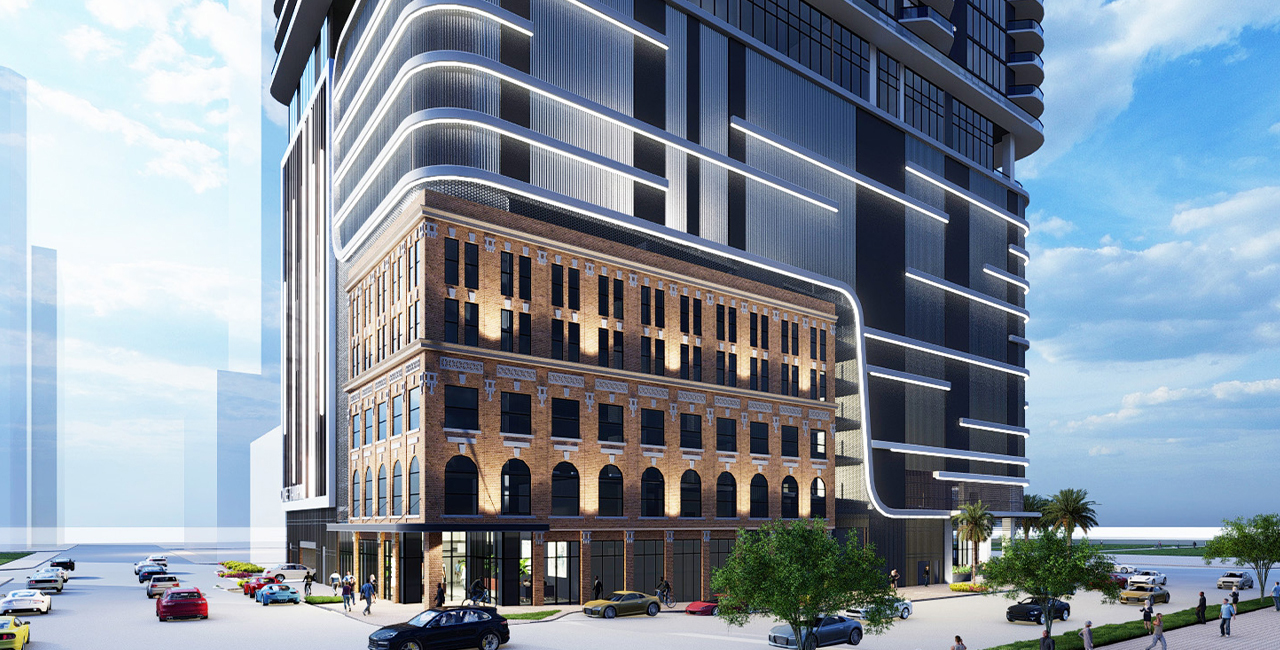This detailed computer-generated image showcases an architectural representation of a futuristic building juxtaposed with a historical structure. The base is a traditional four-story brick building with bottom arch windows and rectangular windows above, exuding an old, historic charm. Atop this historic foundation sits a modern glass skyscraper characterized by its flowing white lines, curved edges, and extensive use of glass, suggesting contemporary condos or flats with balcony spaces.

The scene captures a busy urban environment with a tree-lined boulevard wrapping around the corner of the building. Numerous cars, including sports cars and sedans of various colors, traverse the roads alongside sidewalks filled with computer-generated people, indicating an active community. In the foreground, palm trees add a touch of verdant greenery, hinting at a coastal location. The blue sky, filled with white puffy clouds, forms a serene backdrop, contrasting with the bustling cityscape and merging past architectural styles with futuristic design elements.